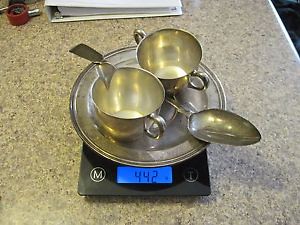In the image, a granite-style countertop serves as the backdrop. On this surface, centered prominently, is a small digital food scale with a circular base and a square display panel reading "442g" in illuminated blue digits. The scale features two buttons, labeled 'M' on the left and 'T' on the right. Positioned on the scale are three sterling silver kitchen items: a cup with two handles, a creamer with a spout and handle, and a silver spoon. These items are meticulously arranged for weighing. In the background, there is a white binder, which could be a recipe book, and to the back left, a red circular object that appears to be a thermometer. The detailed setup highlights the precise weight measurement of these elegant silver utensils against the sophisticated granite-style tabletop.